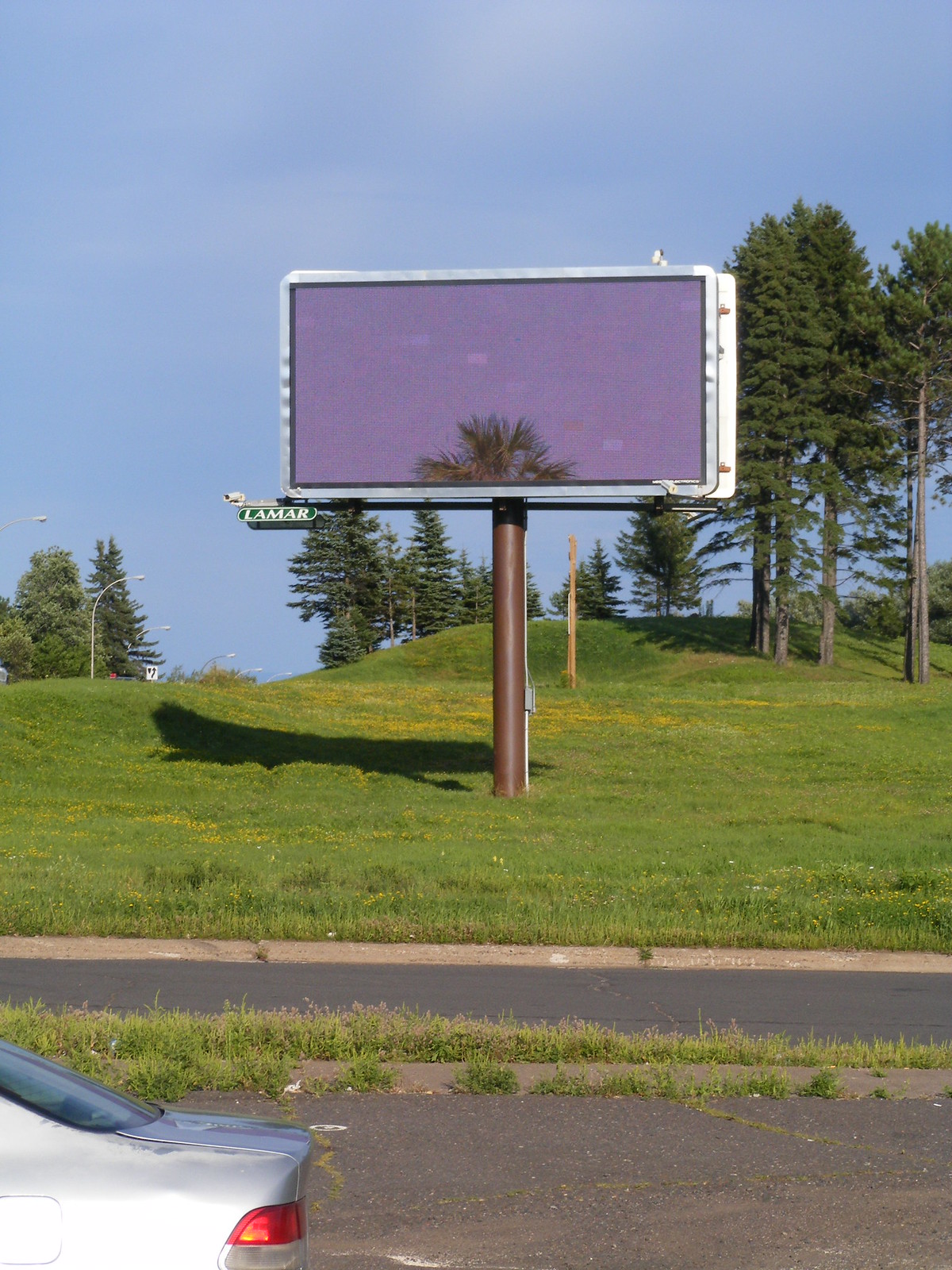The photograph captures a blank billboard situated in a grassy and slightly hilly field, bordered by a few scattered tall pine trees in the background. The image is taken from a vehicle on a road or parking lot, evident from the cut-off rear of a silver sedan with red taillights visible in the lower left corner. The scene is framed with a thin strip of grass leading to another road with a cement curb.

The billboard, mounted on a somewhat rusted, cylindrical post framed in light silver metal, displays a purplish-blue screen. The only notable detail on the board is a small image of the top of a palm tree at the bottom center, alongside a small tag reading "LAMAR" on the lower left, presumably indicating the advertising company. Adding to the scene's tranquility, a bird, likely a seagull, is perched on the right-hand side of the billboard. The grass in the area is manicured yet slightly long, interspersed with tiny white flowers, contributing to a serene rural setting. The photograph is taken during the daytime under clear blue skies, suggesting pleasant weather around 11 a.m.